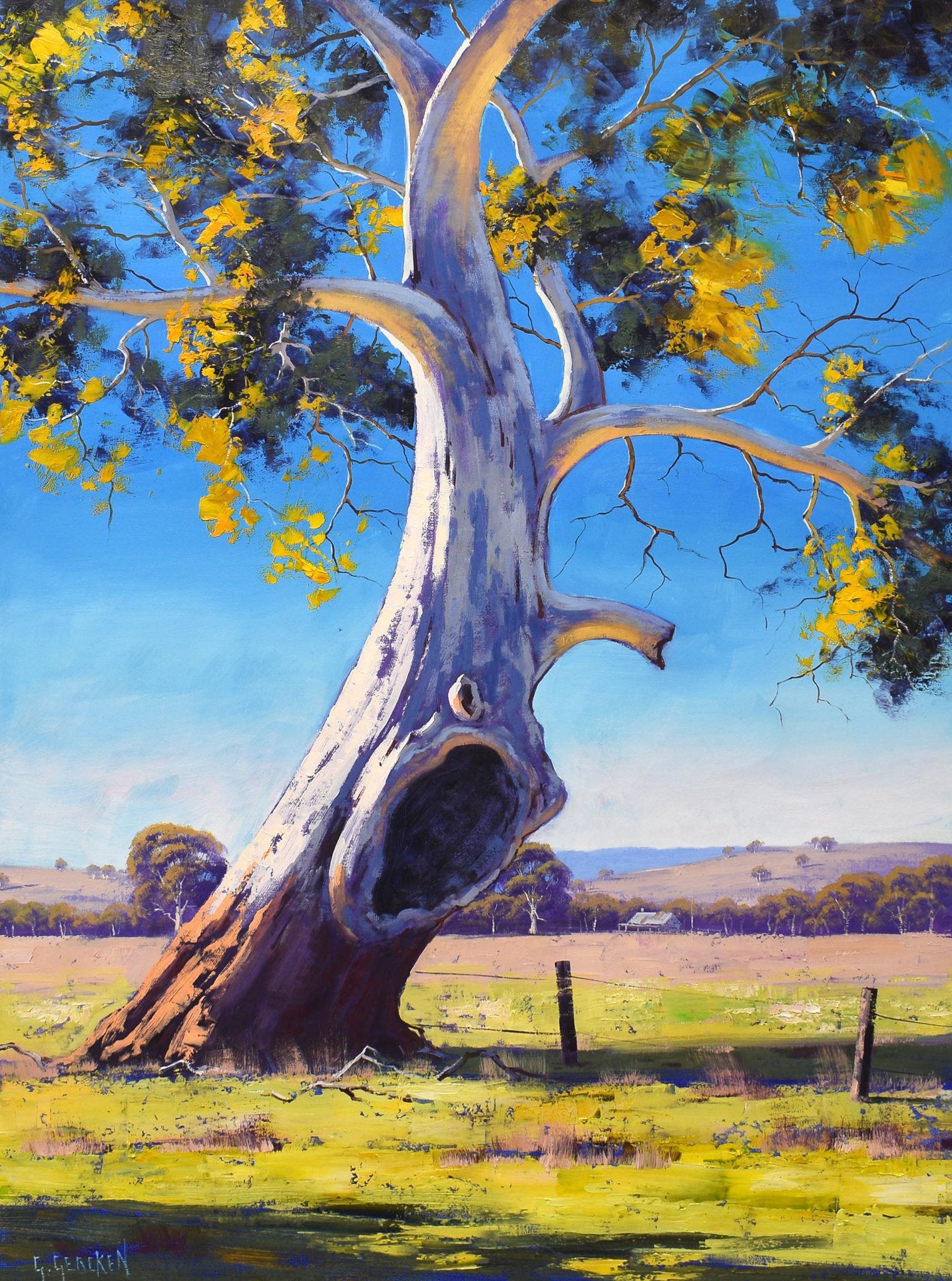This vibrant and somewhat comical painting depicts an outdoor scene centered around an ancient, large tree with curvaceous and expansive branches. The tree is portrayed using shades of brown and gray at its base, transitioning to white at the top, adorned with green and yellow leaves that become darker towards the center of the branches. Notable characteristics include a large hole in the tree's center that resembles an eye, evoking an expressive, almost screaming appearance. Further details include a smaller hole above the main one, enhancing the anthropomorphic semblance of the tree.

In the foreground, the grassy area features hues of lime green and yellow. Adjacent to the tree, a long fence can be seen with visible fence posts, accompanied by small brown sticks in the ground tied with what look like wires or ropes.

The background exhibits rolling hills and a tan field, with the horizon marked by a blue sky transitioning to white with fluffy clouds appearing on the horizon. Off to the right side of the tree, there is a small white house with a white roof, nestled amongst other green-leaved trees with white and brown stems. Additional smaller plants populate the area around the main tree, creating a lively and detailed scene. In the bottom left-hand corner, the artist’s signature "G. Geekin" is visible in white.